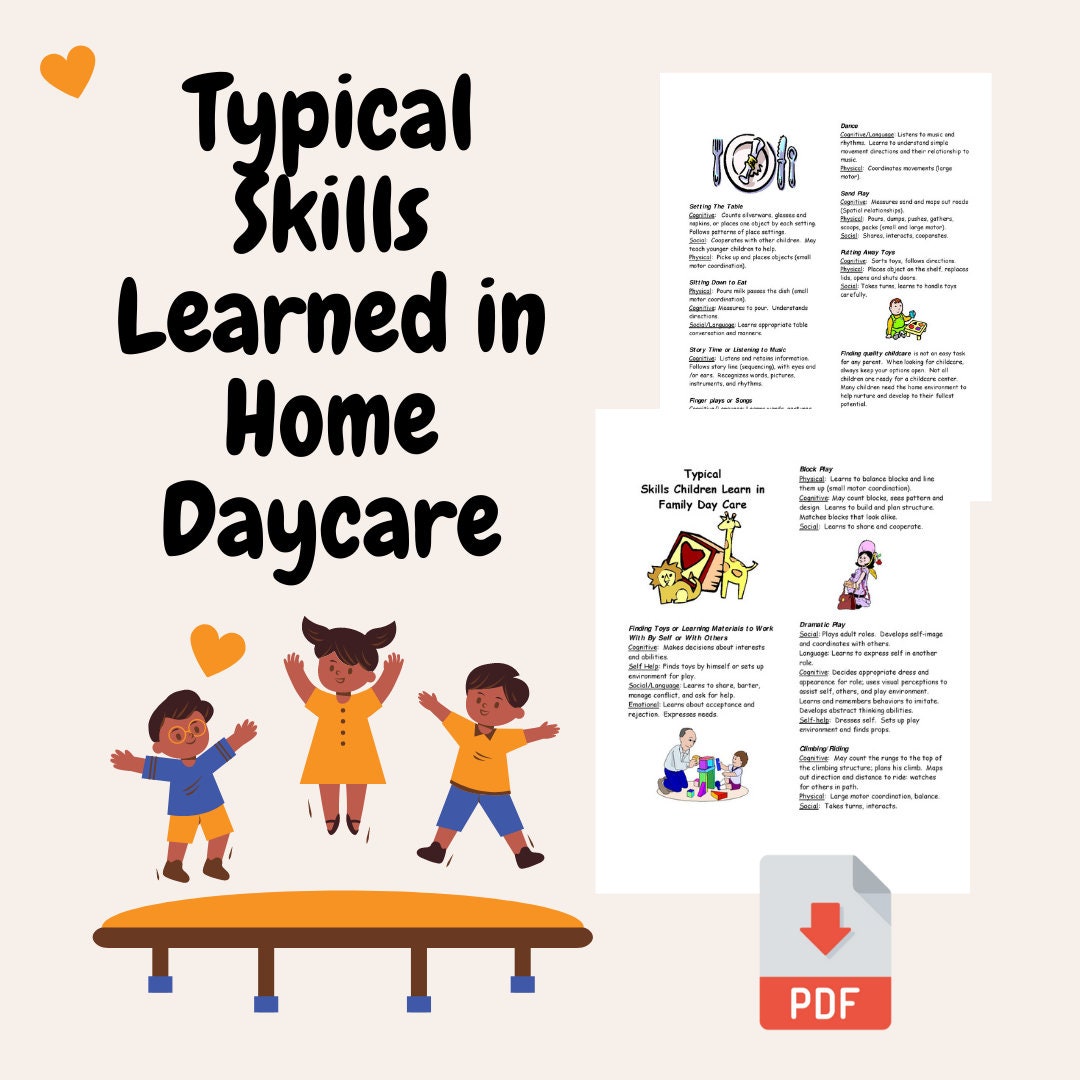This vertical image features a display with a cream to beige background adorned by an orange heart in the upper left corner. Along the left edge in black text, the heading reads: "Typical skills learned in home daycare." Below this, a vibrant illustration depicts three children energetically jumping on a trampoline. The girl, positioned centrally, is dressed in all orange and has brown hair. To her left, a boy wears a blue shirt, orange pants, and brown shoes. On her right, another boy sports an orange shirt, blue pants, and dark shoes. All three children have tanned or brown skin. On the right side of the image, various icons are presented: a plate with silverware symbolizing meals, a block featuring a giraffe and a lion, and an illustration of an adult and a child playing with blocks, representing educational activities. At the bottom, an arrow points downward with the label "PDF," indicating the availability of a downloadable document.